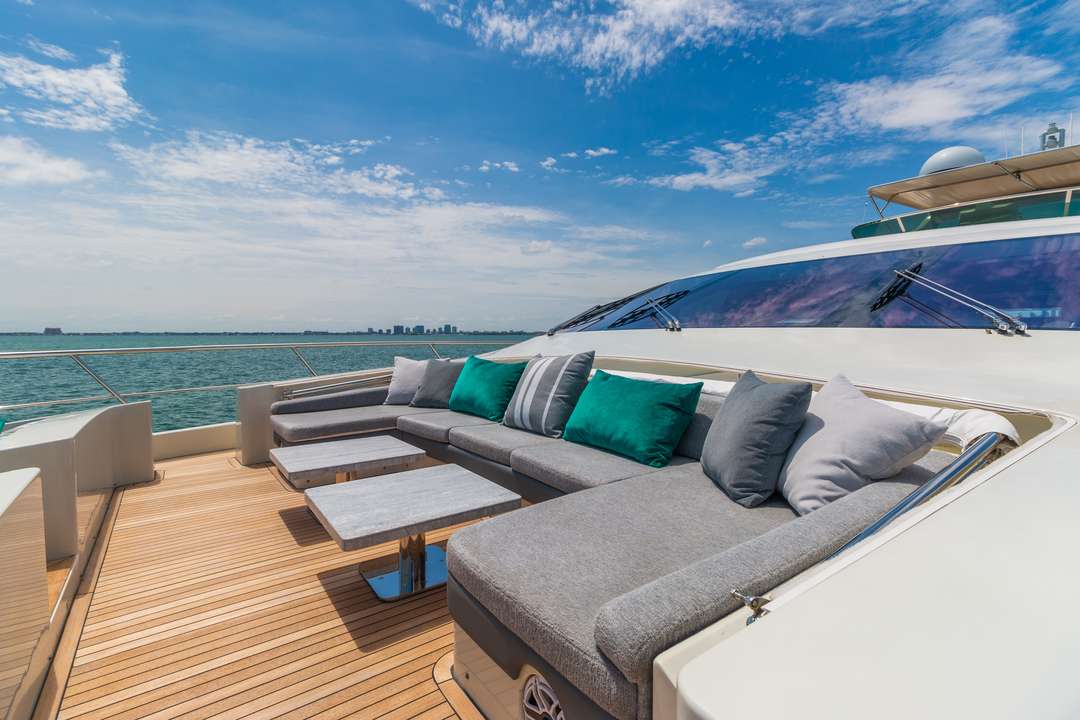This photograph depicts the front deck of a substantial, yacht-sized boat set against the serene backdrop of a blue sky with white clouds and a distant city skyline. The foreground of the image showcases an eye-catching U-shaped lounge area featuring a gray cushioned sofa adorned with an assortment of decorative pillows in shades of green, gray, and white. Positioned in front of the sofa are two sleek, bolted-down coffee tables crafted from metal. The deck's surface is composed of natural wood, which adds a touch of elegance to the outdoor setting and is bordered by a sturdy metal railing designed for safety.

Moving to the rear of this lounge area, the enclosed cabin is visible with its darkened front windshield, equipped with windshield wipers, providing a peek into the cockpit or bridge of the yacht, though the interior remains obscured. To the right, a window allows a slight glimpse into the yacht's interior, possibly hinting at more seating or operational areas. The overall composition of the photograph is completed by the calm, slightly greenish-blue sea in the background, harmoniously blending the luxury of the yacht with the tranquil marine environment.